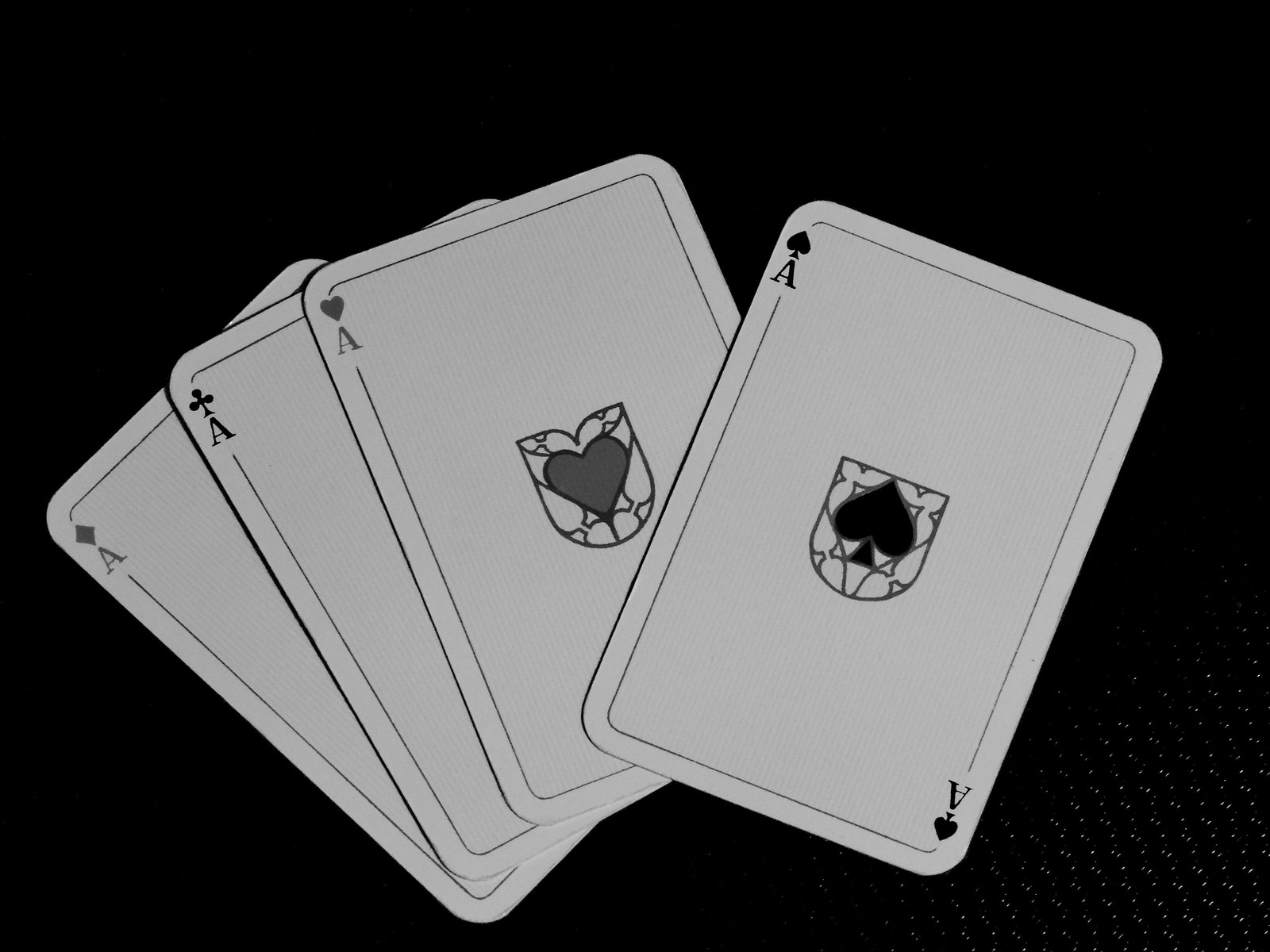In this black-and-white photograph, there are four playing cards, all aces, arranged in a slightly fanned-out stack. The ace of spades is prominently displayed on top, featuring a small spade symbol in the top left corner, a larger spade on a gold shield in the center, and another spade in the bottom right corner. To the left of the ace of spades lies the ace of hearts, followed by the ace of clubs further to the left. The bottom-most card, partially visible with about one-fourth of it showing, is the ace of diamonds. The cards rest on a dark, textured tabletop, with the grain of the surface subtly visible beneath them, adding depth and contrast to the composition.